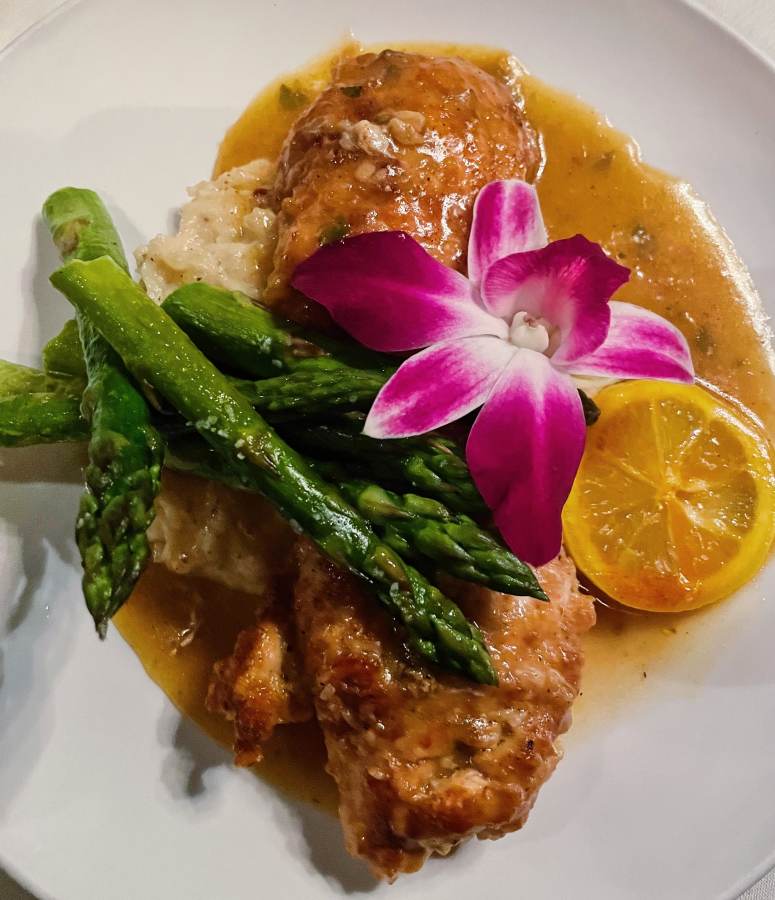This overhead view showcases a beautifully prepared meal on a white plate, featuring a central piece of meat—possibly chicken, pork, or fish—arranged vertically and topped with an elegant pink and white flower as a garnish. The meat is generously covered with a rich sauce or brown gravy. To the right of the meat, there's a slice of lemon or orange bathed in the glaze. On the left, fluffy mashed potatoes peek through, accompanied by several sprigs of asparagus, glistening with either moisture or butter. The composition is tight, with the edges of the plate just visible, emphasizing the intricate presentation of this appetizing dish.